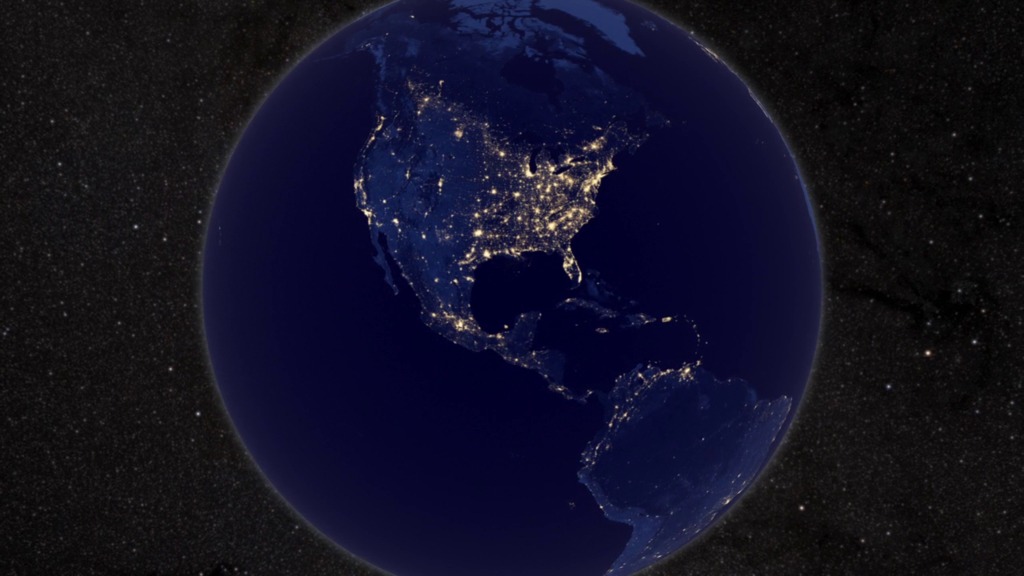The image depicts a mesmerizing outer space view of Earth, showcasing North and South America. At the center, North America is prominently displayed with the United States brightly illuminated, especially along the East Coast. Above lies Canada, and below it, Mexico extends into Central America, touching the top of South America and neighboring the Caribbean islands. The Earth is depicted in rich, dark blues and indigos, bordered by a striking gold ring that adds a touch of ethereal beauty. Sparkly gold dust outlines the countries, giving off a bioluminescent appearance that contrasts with the dark vacuum of space. Tiny white and red stars scattered across the blackness of space accentuate the scene, creating a vivid starry backdrop. The lights from populated areas on Earth highlight the distribution of human habitation, from the densely populated East Coast of North America to the less illuminated regions of Mexico, Central America, and South America.